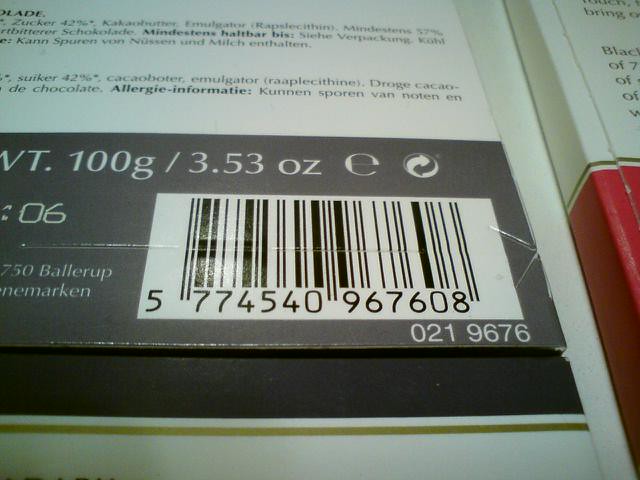This close-up photograph prominently features a UPC barcode on the back of a product's packaging. The primary focus of the image is the barcode, which is situated on gray packaging with white characters. Surrounding the barcode are various elements of the packaging. Above the barcode, there is text providing ingredient information in what appears to be German, accompanied by weight details indicating "100 grams" and "3.53 ounces." To the right of the barcode, there are some iconic symbols and partial address information. Adjacent to the barcode, a second packaging section is visible, characterized by a color scheme with a black base, thin green stripe, and a white top. Below this is another visible section which mirrors the pattern with a black top bar, thin green stripe, and red bottom. The packaging details suggest it is possibly related to allergy medication or another health-related product.